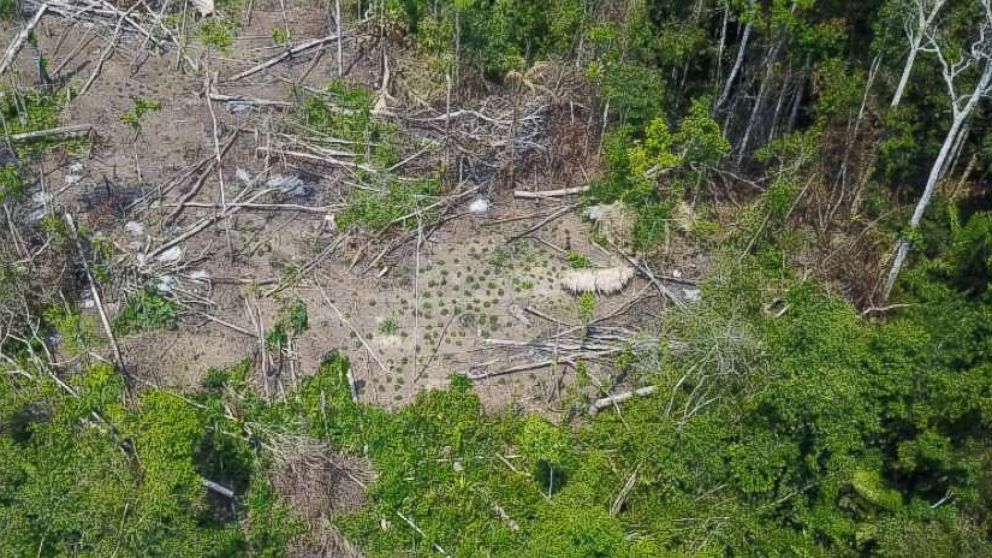This aerial photograph, likely taken from a drone or a low-flying helicopter, captures a striking contrast within a dense forest. At the outer edges of the image, the forest canopy is lush with verdant, green leaves. However, the focus of the image reveals a large, deforested section at the center, where numerous felled trees with white trunks lie haphazardly on the forest floor. The absence of equipment or personnel suggests the logging operation is either paused or completed. The scattered arrangement of the trees indicates they were recently cut and left in place rather than being collected. Patches of light brown dirt, white rocks, and sparse shrubbery intersperse the area, making the disruption to the natural landscape stark and sobering.